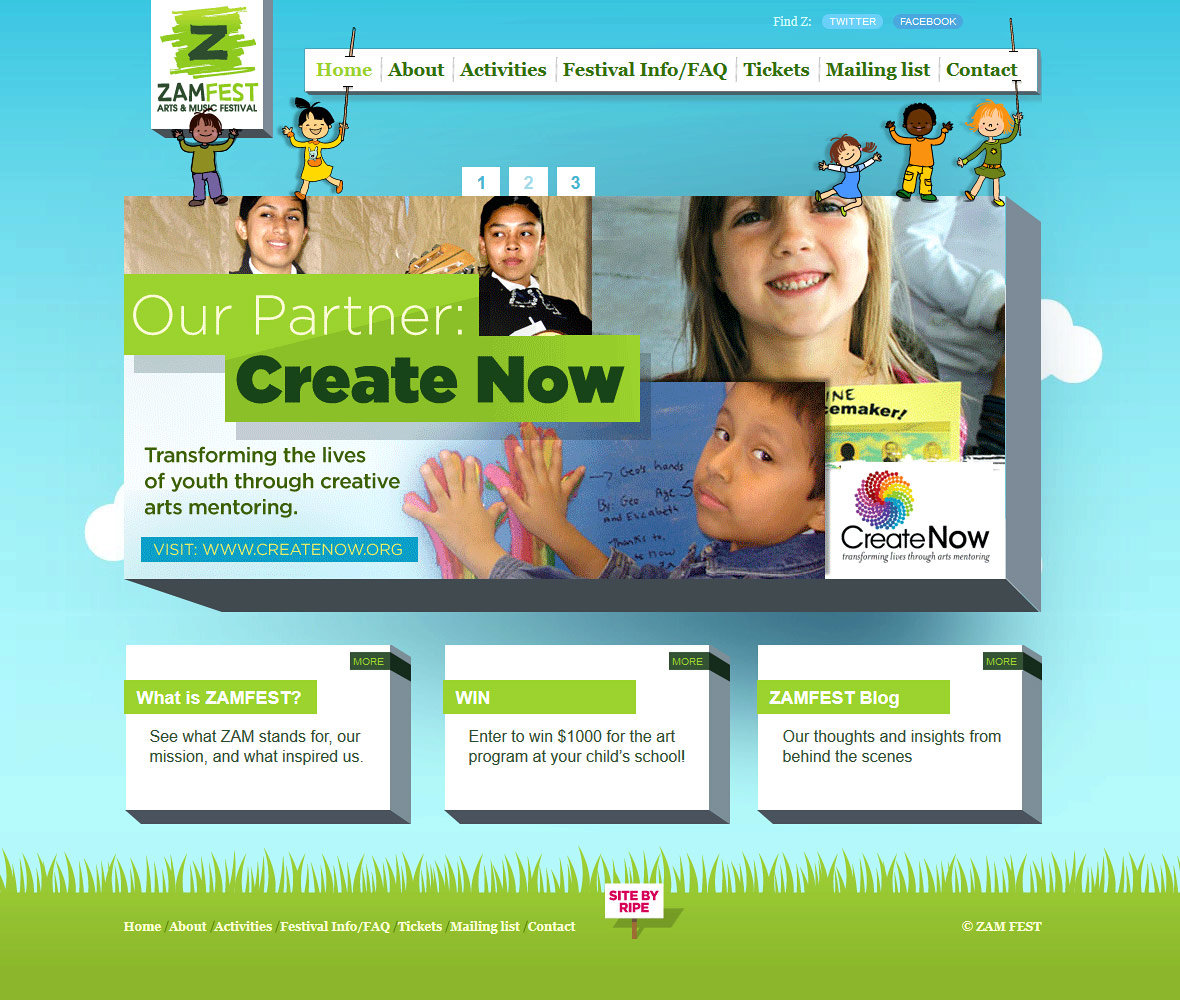The image showcases a promotional flyer for the ZamFest Arts and Music Festival. The flyer features a cartoonish child character holding a sign that reads "ZamFest Arts and Music Festival." The sign is white with a prominent green "Z," artistically outlined with scribble lines forming the background.

The website navigation menu includes the following sections: Home, About, Activities, Festival Info/FAQ, Tickets, Mailing List, and Contact. Below the menu, a banner highlights the festival's partner, 'Create Now,’ accompanied by images of children. One child is depicted with their hands up, engaging with a drawing or possibly a board. 

The banner text reads: "Transforming the Lives of Youth Through Creative Arts Mentoring." Directly beneath this is a call-to-action bar inviting viewers to visit the website www.createnow.org.

At the bottom of the flyer, there are three informational boxes. The first box is titled "What is ZamFest?"